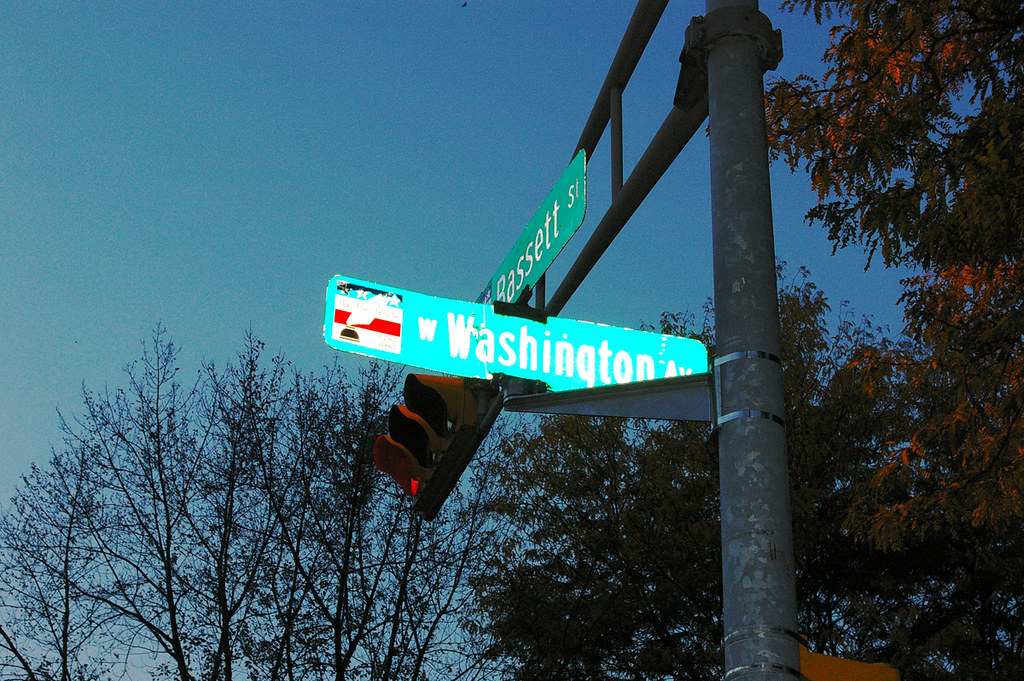This image captures an intersection near dusk, featuring a gray metallic streetlight pole with attached street signs for West Washington Avenue and Bassett Street. The sky is darkening, suggesting early nighttime or late dusk. The glare from the streetlights indicates that a camera flash was likely used. The traffic light on the horizontal arm of the pole shows red. Surrounding the intersection are trees with mixed foliage, typical of early fall—some trees display dense leaves, while others have already shed a portion. The environment suggests a more bustling area rather than a quiet suburban street, with the green and white street signs and yellow-encased traffic signals indicating a well-traveled route.